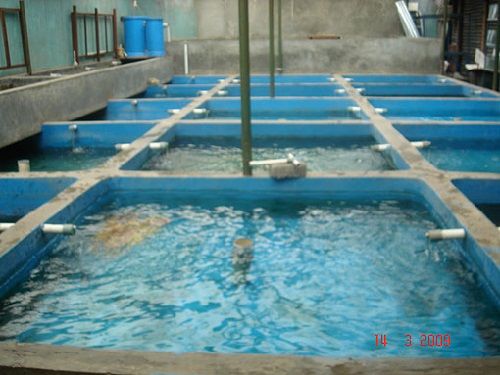This image depicts an indoor water treatment facility or possibly a fish farm, prominently featuring several rows of water tanks or separated pools which dominate the bottom and center of the composition. The tanks are aligned in three rows of five and appear to be integrated into the building's structure. The primary colors visible in the image are various shades of blue, white, grey, brown, teal, orange, red, and black. To the left, a stone or concrete wall can be seen, while the upper right of the image is indistinct and less discernible. The environment has an industrial feel, with some buckets visible towards the back on the left-hand side, adding to the impression of an experimental or processing area. In the bottom right corner, a date—14-3-2009—is displayed in red lettering.